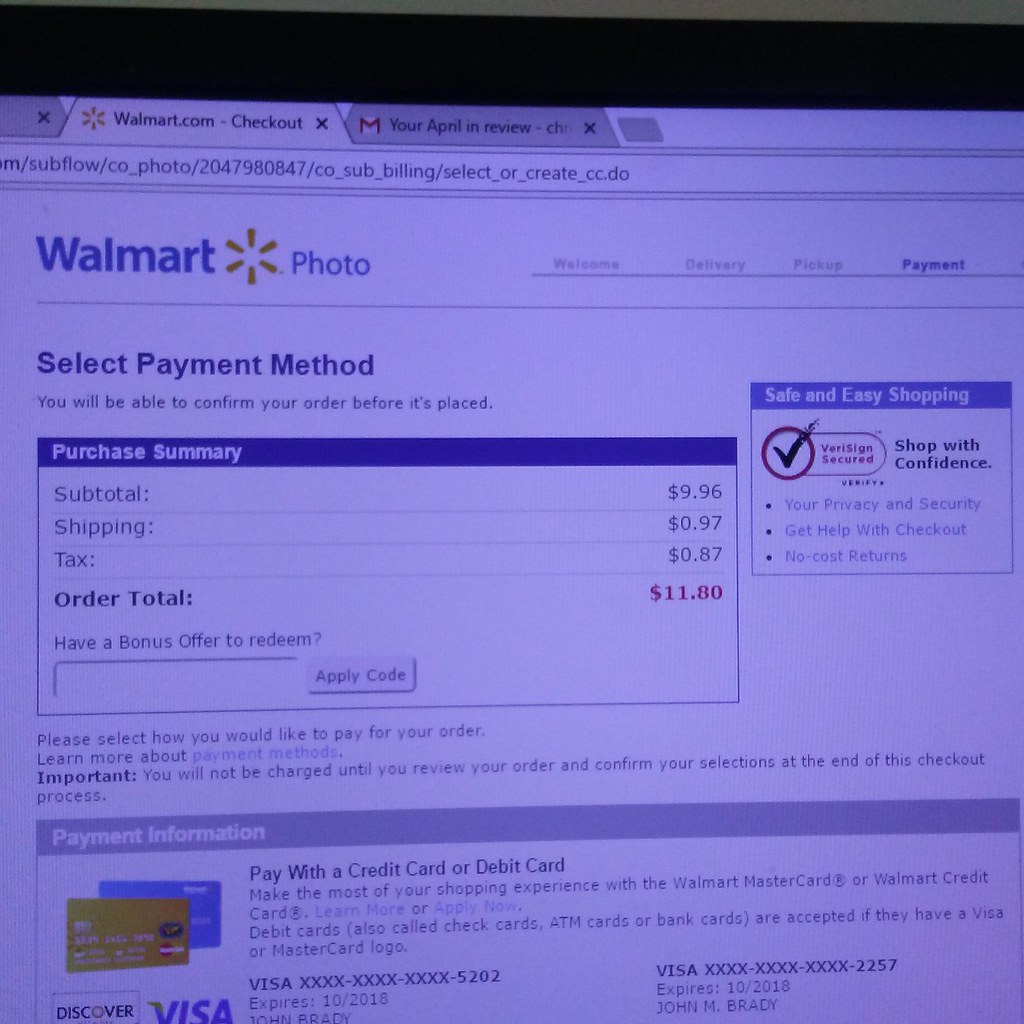The image depicts an online Walmart checkout screen. At the top, there are two tabs, with the current tab displayed in white and the tab to its right in gray. Beneath these tabs, the URL bar reads: "subflow/cophoto/[a series of numbers]/co_billing/select_or_create_cc.do." Further down, the Walmart logo appears in blue, accompanied by the word "photo" also in blue. 

The checkout process is divided into four stages: Welcome, Delivery, Pickup, and Payment, with the current stage highlighted as "Payment." The text "Select Payment Method" is prominently featured in blue. Below this, the total amount due is displayed in purple, amounting to $11.80. There is an option to redeem a bonus code, with a gray button marked "Apply Code" beside it.

On the right side of the screen, a banner with a blue background reads "Safe and Easy Shopping," followed by the assurance "Shop With Confidence." Underneath, additional smaller black text provides further details. At the bottom, the screen displays the section for entering payment information, specifically credit card details, to finalize the purchase.